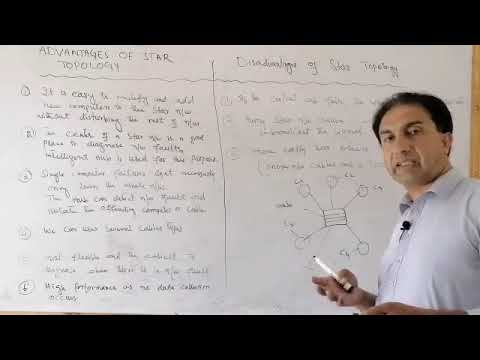The image depicts a middle-aged man, likely a professor or teacher, standing in front of a whiteboard delivering a lecture. He is wearing a light-colored button-up shirt—purported to be a shade of purple or light blue—and has short, dark hair with a receding hairline. A microphone is clipped to his shirt just under his chin. His body faces slightly to the left, while his head is turned to face the camera, showcasing a grimacing facial expression. He holds a dry erase marker in his right hand, poised as if to write.

The whiteboard behind him is divided into two columns filled with black text. The left column is headed "Advantages of Star Topology" and lists multiple bullet points. The right column, titled "Disadvantages of Star Topology," has fewer bullet points and features a diagram beneath the text. The edges of the image are framed by horizontal black bars at the top and bottom, and the professor's left shoulder is partially out of frame on the left side.